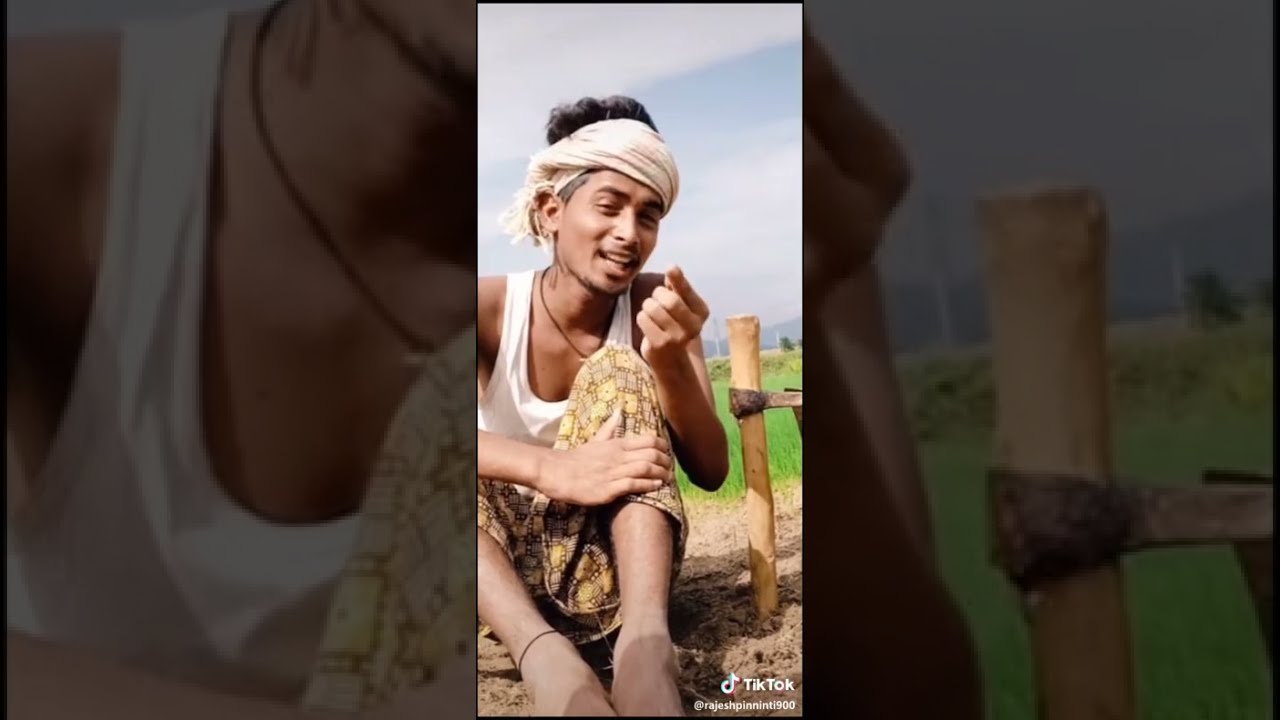In this TikTok image, a man of Asian descent is captured sitting on the ground during the daytime, his surroundings marked by a noticeable dusty and grassy area. He is positioned in front of a green field, with a light blue sky scattered with white clouds overhead. The man is thin, wearing a white tank top paired with loose, baggy yellow and brown pants, and has bare feet. An off-white cloth is wrapped around his head, allowing some of his dark brown hair to peek through, and he sports a small beard. He appears to be either smiling or in the middle of speaking. A small wooden fence stands to his right. The image is a horizontal rectangle encompassing a vertical TikTok video, with the TikTok logo and the handle "@rajshippingnint900" visible in the bottom right corner.